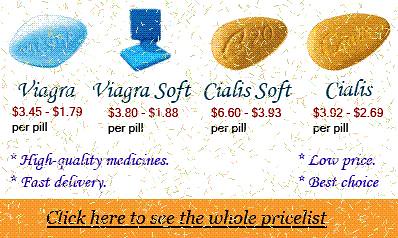The image has a white background with a small band of orange across the bottom, scattered with confetti. Along the bottom, black text underlined in orange reads "click here to see the whole price list," though it's somewhat hard to read. The central focus is on four different varieties of erectile dysfunction pills displayed in the upper portion. The first pill is blue, labeled Viagra, priced between $3.45 and $1.79 per pill. To its right is Viagra Soft, also blue, priced slightly higher at $3.80 to $1.88 per pill. Next is Cialis Soft, an orange egg-shaped pill, with a range from $6.60 to $3.93 per pill, making it the most expensive. Lastly, there is Cialis, priced between $3.92 and $2.69 per pill. In blue and purple text, promotional slogans highlight "high quality medicines, fast delivery, low price, best choice."